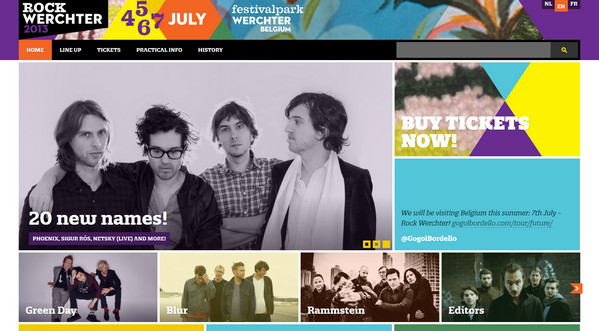Here is a cleaned-up and detailed caption for the image:

---

The Rock Werchter 2013 music festival website, promoting the event held between July 4th and 7th at Schiphol Park in Werchter, Belgium. The homepage highlights various features such as a "Buy Tickets Now" button, social media links, and options to change the site's language. Dominating the page is a main image announcing "20 New Names" including Phoenix, Sigur Rós, Metric, and more, alongside visuals of bands like Green Day, Blur, Rammstein, and Editors. Each band is represented with a photograph, predominantly showcasing white male rock musicians. The interface also includes a search bar in the top-right corner, as well as navigation links directing to sections on the lineup, tickets, practical information, and the festival's history.

---

This caption maintains the original details while presenting them in a more structured and coherent manner.